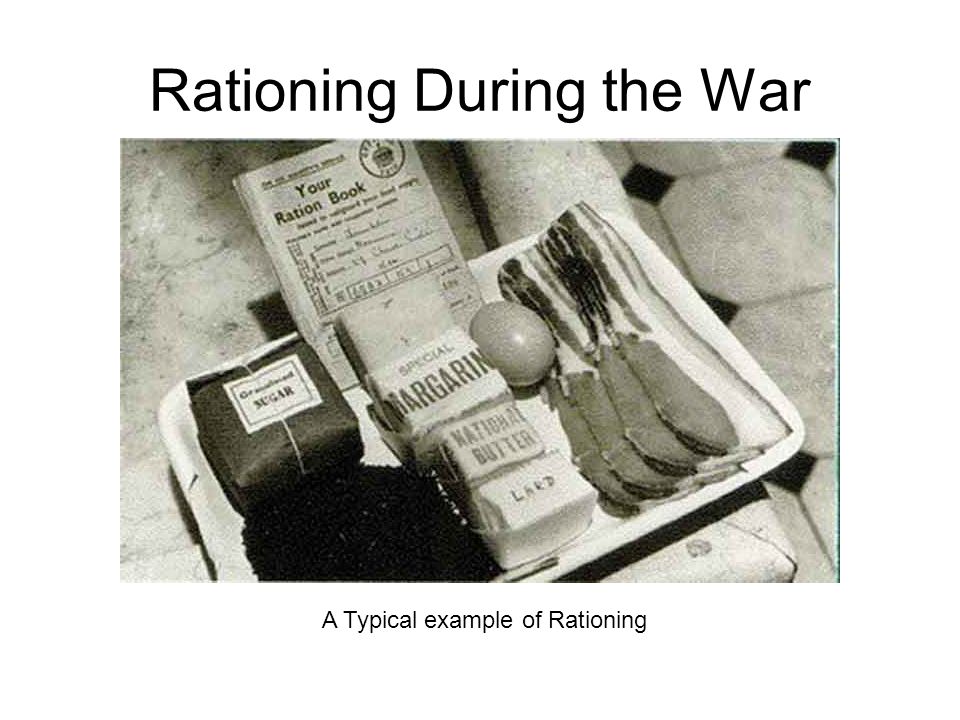The image, titled "Rationing During the War" in large sans-serif font with a subtitle "a typical example of rationing," is a weathered black-and-white photograph, likely from World War II or the Korean War, presented as a slide. The photograph shows a tray of various rationed food items set against a tiled background. At the top of the tray is a partially readable booklet labeled "Your Ration Book." On the top left lies a square package labeled "granulated sugar." Centrally positioned from top to bottom are partial sticks of margarine, national butter, and lard. To the right of these, a single egg is visible. Also on the tray, somewhat to the right, are strips of bacon with four more indiscernible strips of perhaps another type of meat on top. In the bottom left corner of the tray sits a dark object, its identity unclear. The ration book appears to have a stamp in the top right corner, though the details of the stamp are illegible.